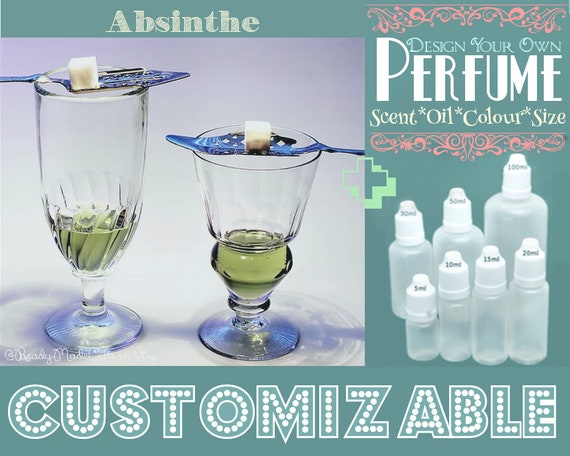The advertisement features a muted teal background divided into two sections. On the left, there is an inset color photograph depicting two clear glasses, each filled about a quarter with a green liquid, signifying absinthe. A metallic, likely silver, absinthe spoon rests crosswise on top of each glass, holding a white sugar cube. Above the photo, in light green text, reads "ABSINTHE." The right section of the ad, on the teal backdrop, promotes the customizable nature of perfume creation. In white, art-deco styled text, it states "DESIGN YOUR OWN PERFUME" with smaller decorative text listing "scent, oil, color, size" in beige font. Accompanying this text is an image of empty, clear plastic bottles with white caps, arranged by size from five milliliters to 100 milliliters. Along the bottom, a white marquee-style typeface reads, "CUSTOMIZABLE," emphasizing the bespoke nature of the product. The ad is framed by red filigree borders at the top and bottom, enhancing its visual appeal.